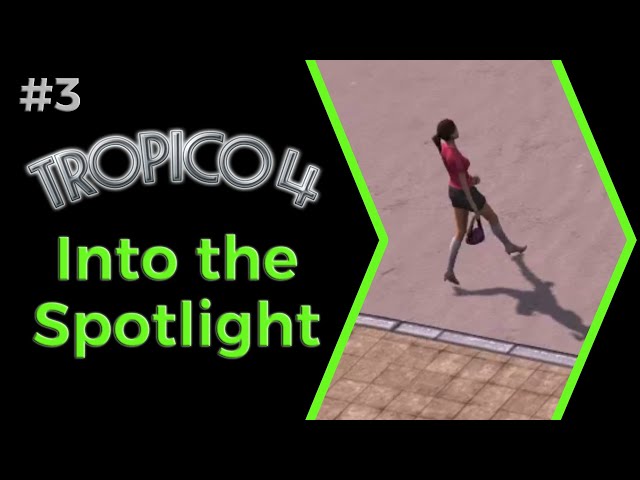The image features a flat, perfectly black background, resembling a PowerPoint slide. In the top left corner, the text "#3" is displayed in a silver metallic color. Below that is the curved text "Tropico 4" in the same metallic hue, followed by the phrase "Into the Spotlight" in green. To the right, a wide arrowhead shape points to the right, forming a cutaway that reveals an in-game street scene. The scene is sunny, casting a clear shadow of a woman walking on a plain concrete street with a tiled sidewalk beside her. She has a black ponytail and is wearing a pink or red top, and shorts or a skirt, complemented by high boots. She carries a handbag in her right hand. The visual and text elements combine to create a striking promotional image for Tropico 4.